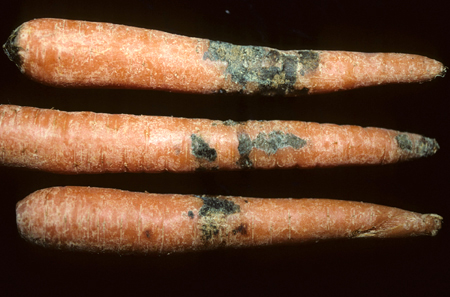The image is a high-resolution photograph of three full-size carrots aligned horizontally against a solid black background, devoid of any borders or text. The carrots are positioned one above the other, with their thick green-top removed ends on the left and their pointed tips on the right. The top carrot, which is the most affected by rot, has a substantial green and black moldy area near its center, accented by smaller white splotches along its length. The middle carrot, partially cut off on the left side of the image, exhibits mold in two locations: a vertical band near the center and additional spots towards its pointed tip. The bottom carrot also displays signs of decay with a darker green mold patch situated slightly above its midpoint, along with scattered white discolorations. The overall appearance of the carrots indicates significant aging, as they exhibit a pale orange hue interspersed with mold and dried textures.